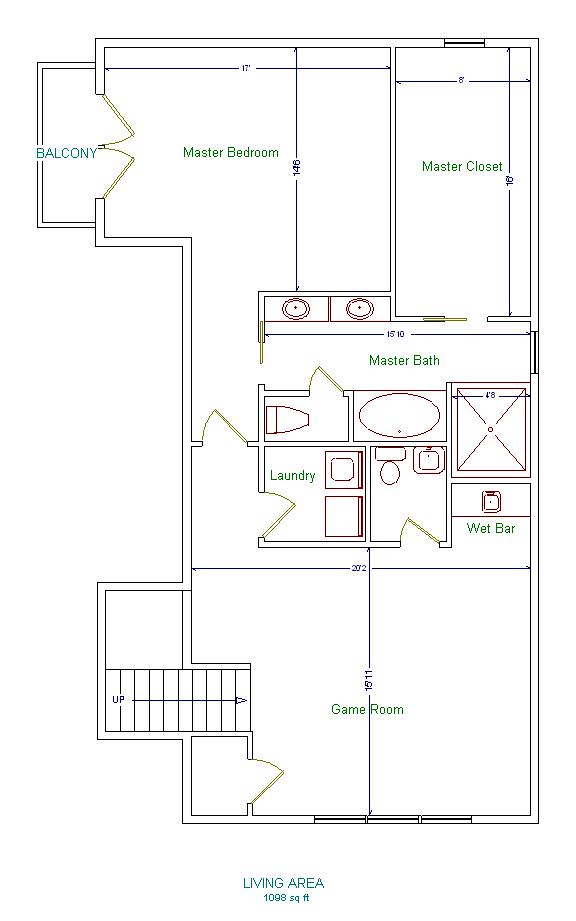**Detailed Caption:**

This is a detailed floor plan of a home's interior, providing a comprehensive layout of the various rooms and their dimensions. The entire diagram, measuring approximately 1098 square feet, is presented from a top-down perspective, with the living area prominently labeled at the bottom of the page.

Starting from the top left, the floor plan indicates a balcony with a small doorway leading into the master bedroom. The dimensions of each room are marked with numerical values on the walls. Adjacent to the master bedroom is a line demarcating the separation from the master closet, which also has detailed measurements annotated.

Directly beneath the master closet is a bathroom sink, followed by a master bathroom, all intricately labeled with doorways and proper walkways. Further down the page, there is a hallway leading to the master bathroom, providing easy access from various parts of the home.

Progressing downwards, the next segment of the floor plan features a laundry room, clearly illustrated with pictograms of a washer and dryer, and the label "Laundry" next to them. Adjacent to the laundry room is a wet bar area.

A stairway is shown beneath these sections, with an indication that it leads upwards. This stairway opens into a small square area that transitions into a game room. The game room is a significant part of the floor plan, with vertical and horizontal lines marking its dimensions and a large doorway at the bottom, allowing for easy access. Various smaller doorways are also indicated throughout the game room for efficient movement within the house.